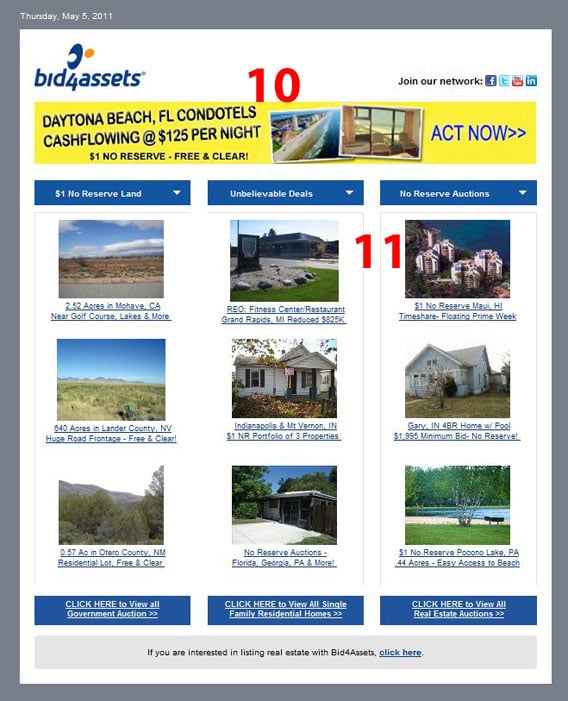A promotional flyer featuring a distinct dark gray border that frames the entire design. The interior is predominantly white, creating a striking contrast. In the top-left corner, the date "Thursday, May 5th, 2011" is prominently displayed. Directly below it, the headline "Bid for Assets" draws attention. 

A vibrant red rectangle containing the phrase "Join our Network" is positioned to catch the eye, flanked by several social media icons encouraging connectivity. Beneath this, a bold yellow rectangle announces: "Daytona Beach, Florida Condo Hotels - Cash Flowing at $1.25 per Night - $1 No Reserve, Free and Clear - Act Now."

The bottom section showcases a grid of nine enticing small images, arranged neatly in three rows of three. Each image highlights either a piece of land or a house. Accompanying each picture are three distinct tags that read "$1 No Reserve Land," "Unbelievable Deals," and "No Reserve Auction." 

Additionally, each image is paired with a clickable link inviting viewers to read more detailed descriptions.